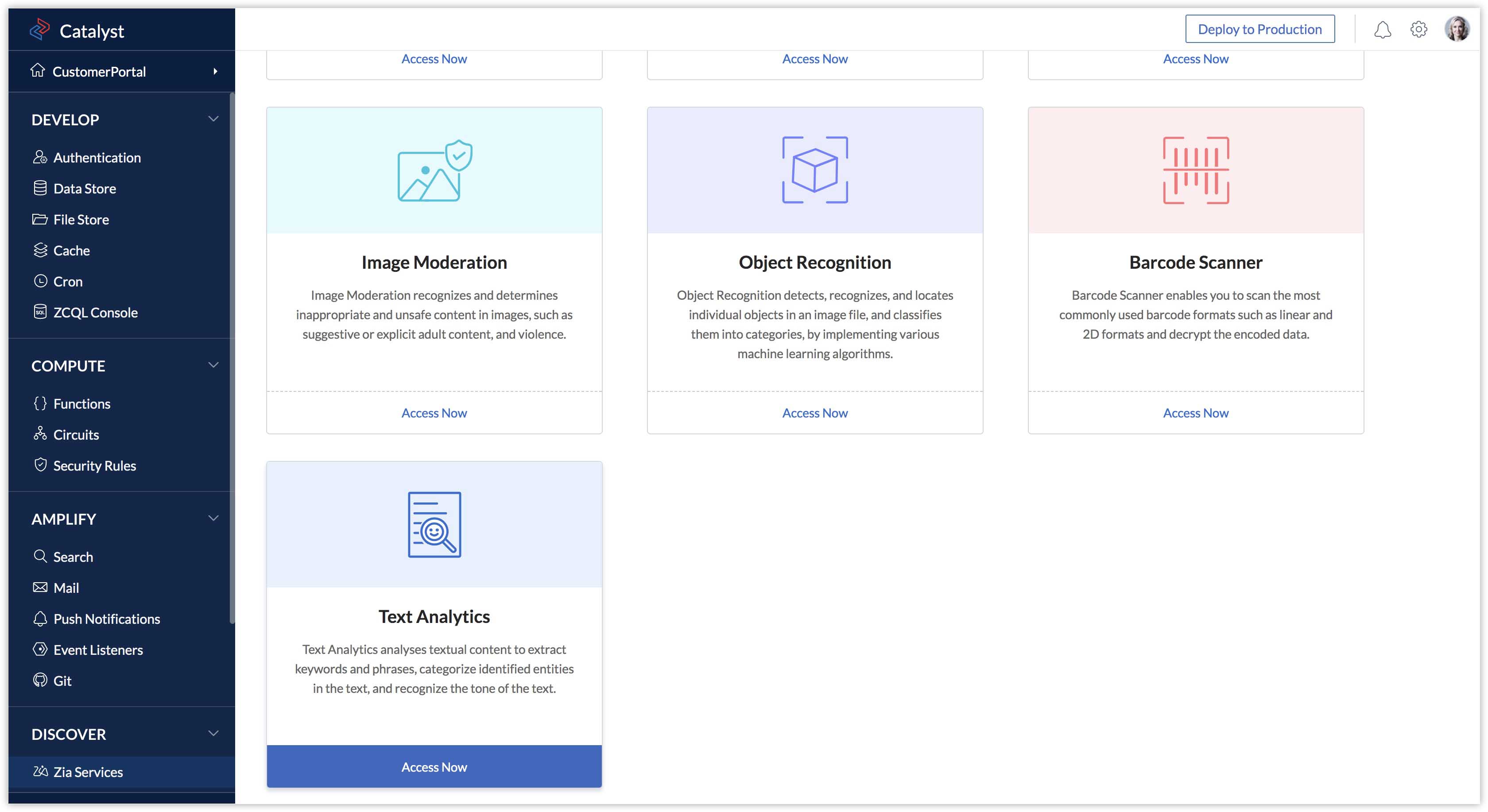**Catalyst Company Web Page Overview:**

On the Catalyst company web page, there is a prominent vertical banner positioned on the left side of the screen. This banner is navy blue and takes up a significant portion of the screen's height. 

- **Banner Details:**
  - At the top left corner of the banner, the word "Catalyst" is displayed in bold white text.
  - Directly below, the word "CustomerPortal" is listed as a single, concatenated word with an arrow pointing right, suggesting navigation to a different section.
  - Further down, the word "DEVELOP" is written in all caps and white text.
  - Below "DEVELOP," there is a vertically aligned list of items including:
    - Authentication
    - Data Store
    - File Store
    - Cache
    - Cron
    - Z C Q L Console
  
- **Additional Categories:**
  - The next category is titled "COMPUTE" with the following items:
    - Functions
    - Circuits
    - Security Rules
  - The third category is labeled "AMPLIFY," listing:
    - Search
    - Mail
    - Push Notifications
    - Event Listeners
    - Get
  - The final category shown is "DISCOVER," under which "Zia Services" is listed.

To the right of the banner, the rest of the screen has a clean, white background with several content boxes, each detailing different functionalities offered by Catalyst, complete with descriptive blurbs and graphics.

- **Functionality Boxes:**
  - **Image Moderation:**
    - This box features a light green, mint-colored ribbon across the top.
    - "Image Moderation" is written in black text beneath the ribbon.
    - The description reads: "Image moderation recognizes and determines inappropriate and unsafe content in images such as suggestive or explicit adult content and violence."
  - **Object Recognition:**
    - This box has a light blue banner at the top.
    - "Object Recognition" is in black text below the banner.
    - The description states: "Object recognition detects, recognizes, and locates individual objects in an image file and classifies them into categories by implementing various machine learning algorithms."
  - There are two more boxes following the same layout principles, each explaining additional functionalities provided by Catalyst. 

This detailed and organized structure makes navigation intuitive, providing users with comprehensive information about the services Catalyst offers.